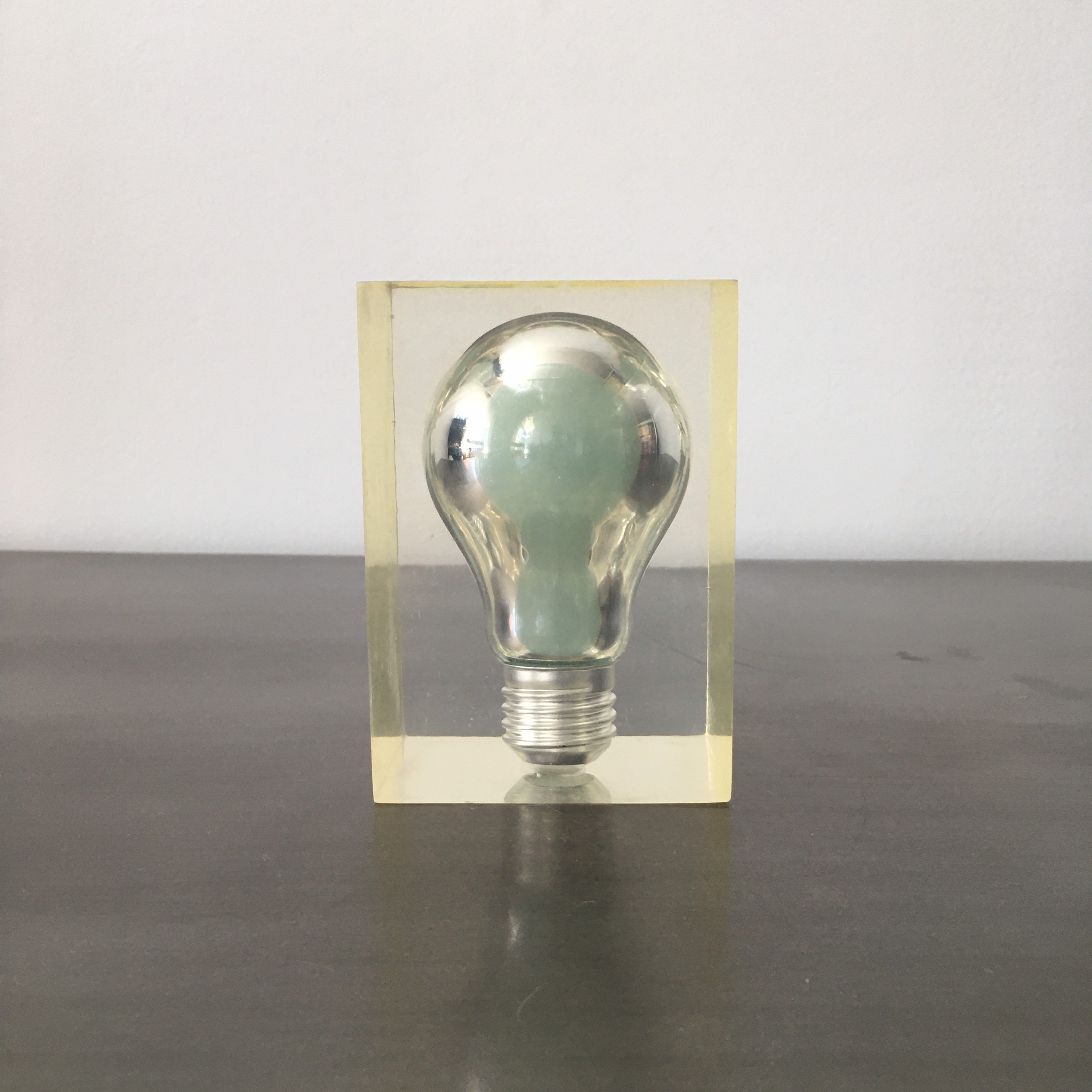The image depicts a single lightbulb positioned at the center, suspended within a translucent, yellow-tinted rectangular stand. The lightbulb appears metallic and reflective, with its silvery surface mirroring hints of light bluish, white, and black reflections. The lightbulb, with a wider top and a narrower, curved base, stands vertically upright on a blackish-brown countertop. The background features a stark white wall, hinting at an indoor setting, possibly within a room or house. No text is present in the image. The scene's lighting suggests some natural light, possibly from a window, reflecting on the bulb’s surface, adding a dynamic interplay of light and shadow. This clear, detailed photograph emphasizes the lightbulb’s sleek form and reflective qualities, sharply contrasting against the simple, neutral-toned backdrop.